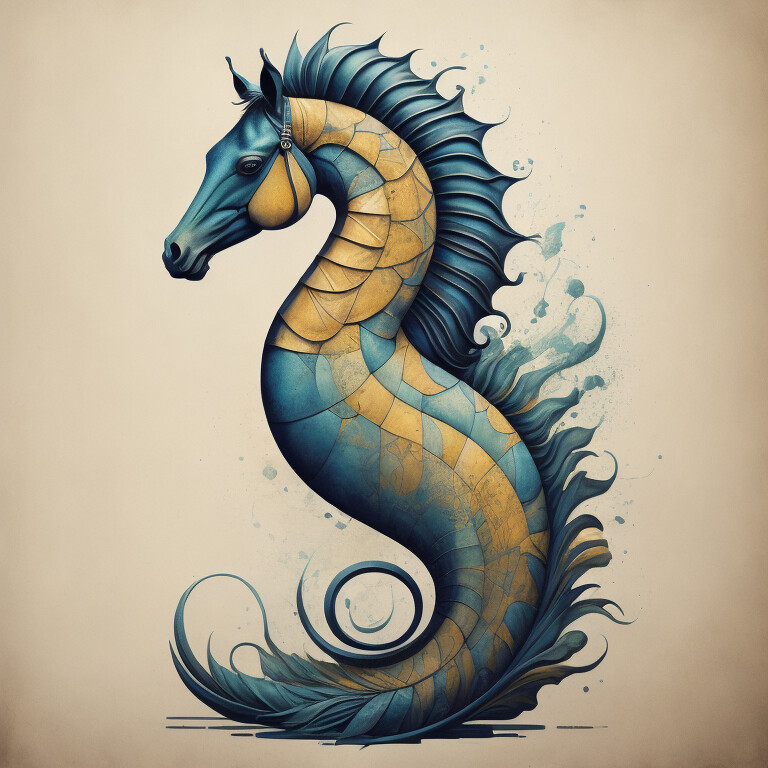The graphic illustration portrays a hybrid creature combining elements of a seahorse and a land horse set against a light brown, almost grayish background. The head closely resembles that of a real horse, complete with blue ears, a long blue nose, and a bridle-like accessory. Its mane, mimicking the texture of fins, runs down the entirety of its serpentine, scaly body. The neck features brown or golden scales interlaced with blue, transitioning into wavy yellow and blue scales along the body. The tail of the creature curls upwards, ending in feathery appendages, and there's a clear shadow below the seahorse on the ground. The entire composition includes elements like splashes and swirls of blue in the background, adding to the visual complexity. The overall scene is vividly detailed, with a focus on the intricate scales and the transformative junction where the horse head blends into the seahorse body. There is no text in the image.